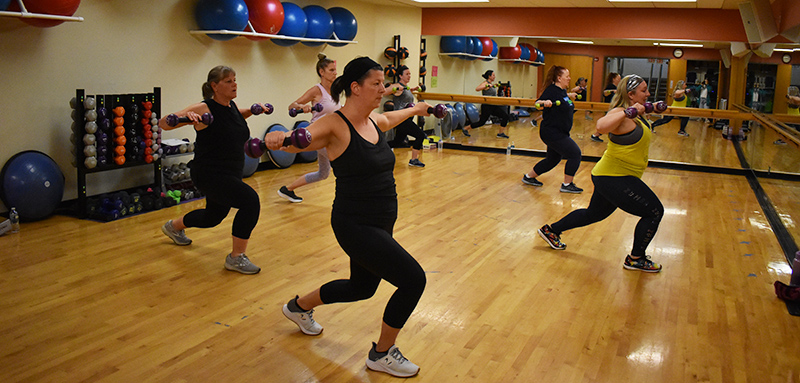In this detailed photograph of a fitness studio, six women are engaged in a coordinated exercise routine, lunging forward with their right leg and lifting weights toward their shoulders. The studio features mirrors along two walls, each with a stretching bar running horizontally across the middle. The space is well-equipped, with a selection of kettlebells on the back wall, hand weights and BOSU balls neatly lined up, and exercise balls stored on a high rack. The women are diverse in build, ranging from thinner to heavier set, and are dressed mostly in black athletic apparel. Notably, one woman sports a bright yellow tank top, while another stands out in a white shirt and purple pants. Their reflections amplify the sense of activity and movement within the room.